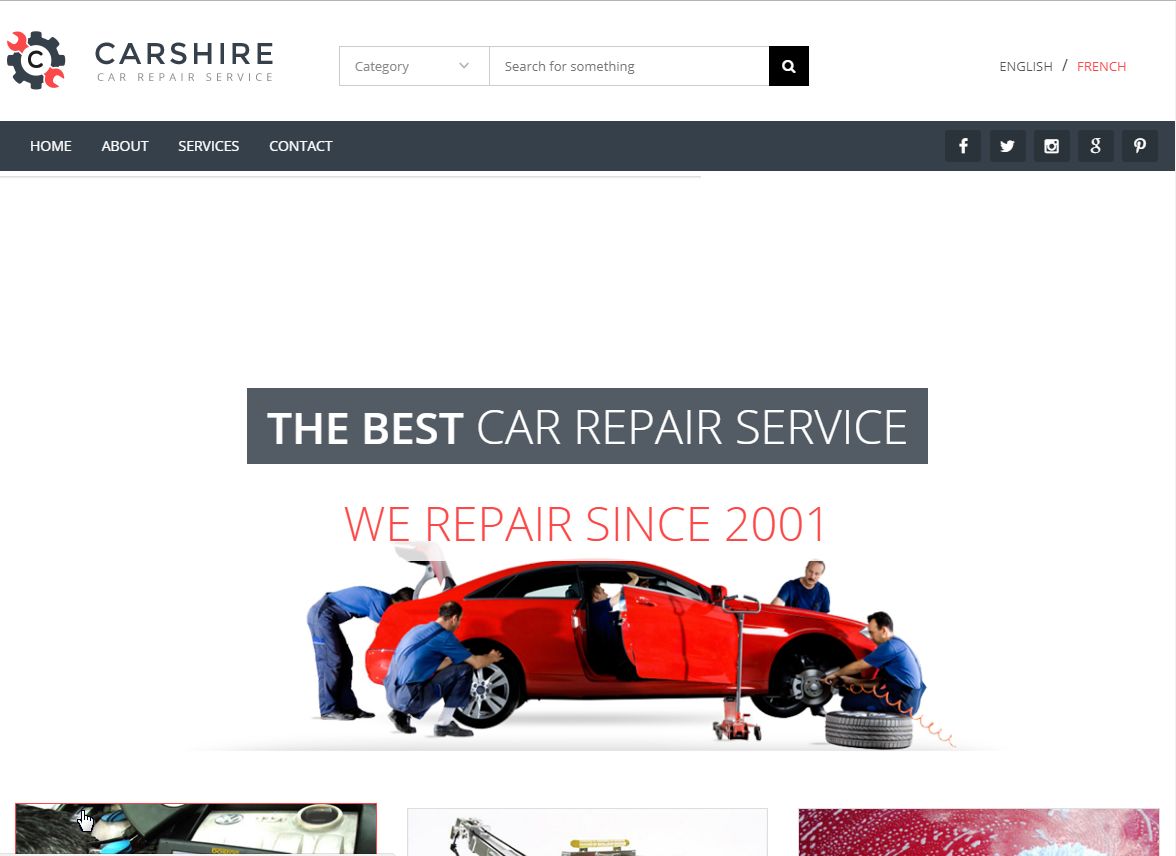This image depicts the homepage of a car repair service website named "CarShire." In the top left corner, the logo features a red wrench with a black tire underneath it, with the letter "C" positioned above the wrench. The logo is complemented by the text "Car Repair Service" beside it.

The top banner consists of a search bar that allows users to choose a category or enter a manual search term. To the right of the search bar, there are language options for English and French, with French highlighted in red. Directly below the top banner is a navigation bar displaying options like Home, About, Services, and Contact. This bar is black with a subtle hint of blue.

Underneath the navigation bar, there's a prominent banner image with large text stating, "The Best Car Repair Service," followed by subtext in red that reads, "We repair since 2001." This section also includes a photo of a red car surrounded by several workers dressed in blue uniforms, actively engaged in repairing the vehicle.

Further down, the page showcases a gallery-like section with three partially visible images, which could potentially serve as links to specific articles or services. The overall design of the webpage is clean and minimalistic, featuring a black-and-white color scheme.